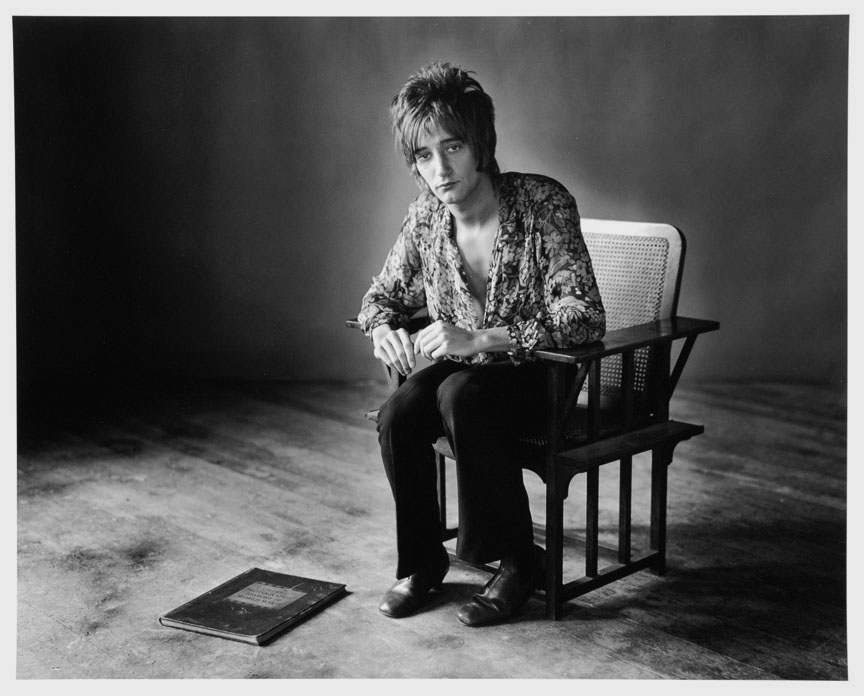The black and white photograph captures a young man, possibly Rod Stewart in 1968, seated in the center of the frame on a brown wicker chair with tall, flat arms. The man looks distinctly uncomfortable as he rests both hands on the chair's armrests, fingers barely touching. He is dressed in a long-sleeve, open-front paisley shirt, exposing part of his chest, paired with black pants and dark-colored leather shoes with squared ends. The setting is indoor, featuring a solid, undistinguished background wall and light-colored wooden plank flooring. In the bottom left of the image, a thin book with a dark cover and an illegible white label can be seen lying on the floor, appearing to possibly be a journal or notebook. The photograph is bordered by a light gray frame, enhancing its portrait-like quality.